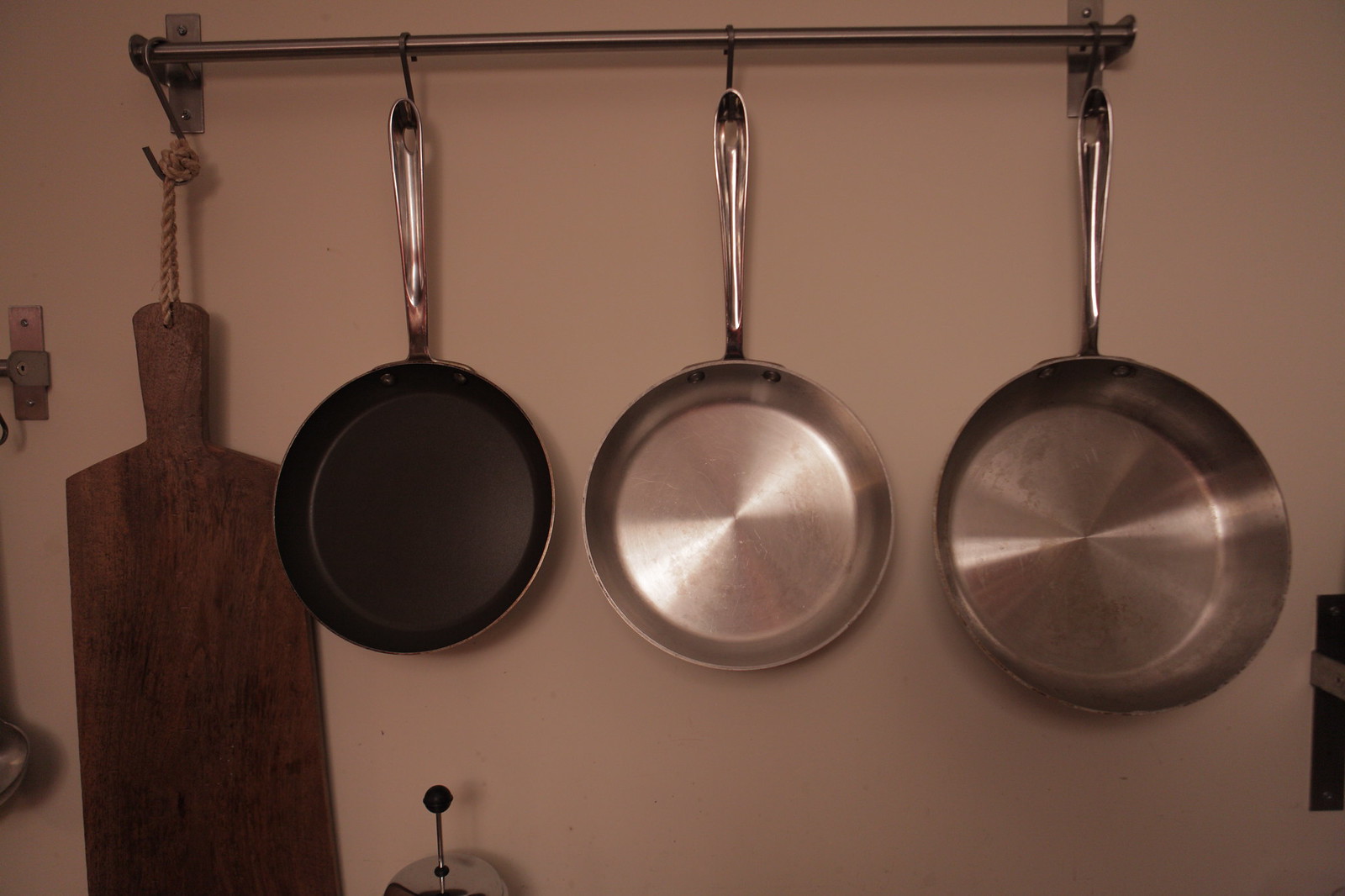In a cozy kitchen with a white, slightly dim background, a metal rod with hooks is mounted on the wall, supporting an arrangement of cookware and utensils. From left to right, a wooden chopping board, resembling a paddle, is secured with a piece of rope, followed by three sauté pans hanging in ascending order by their handles. The first is a black nonstick pan, then a medium-sized stainless steel pan, and finally, a large silver pan with deep sides. The handles of all the pans are of a similar design, extending outward in a straightforward fashion. Just below this arrangement, the top of what appears to be a French press peeks into view. Additionally, off to the side, a smaller rod holding a giant spoon can be glimpsed. The entire scene is captured in a sepia tone, giving it a warm, nostalgic feel with a golden, bronzy finish.